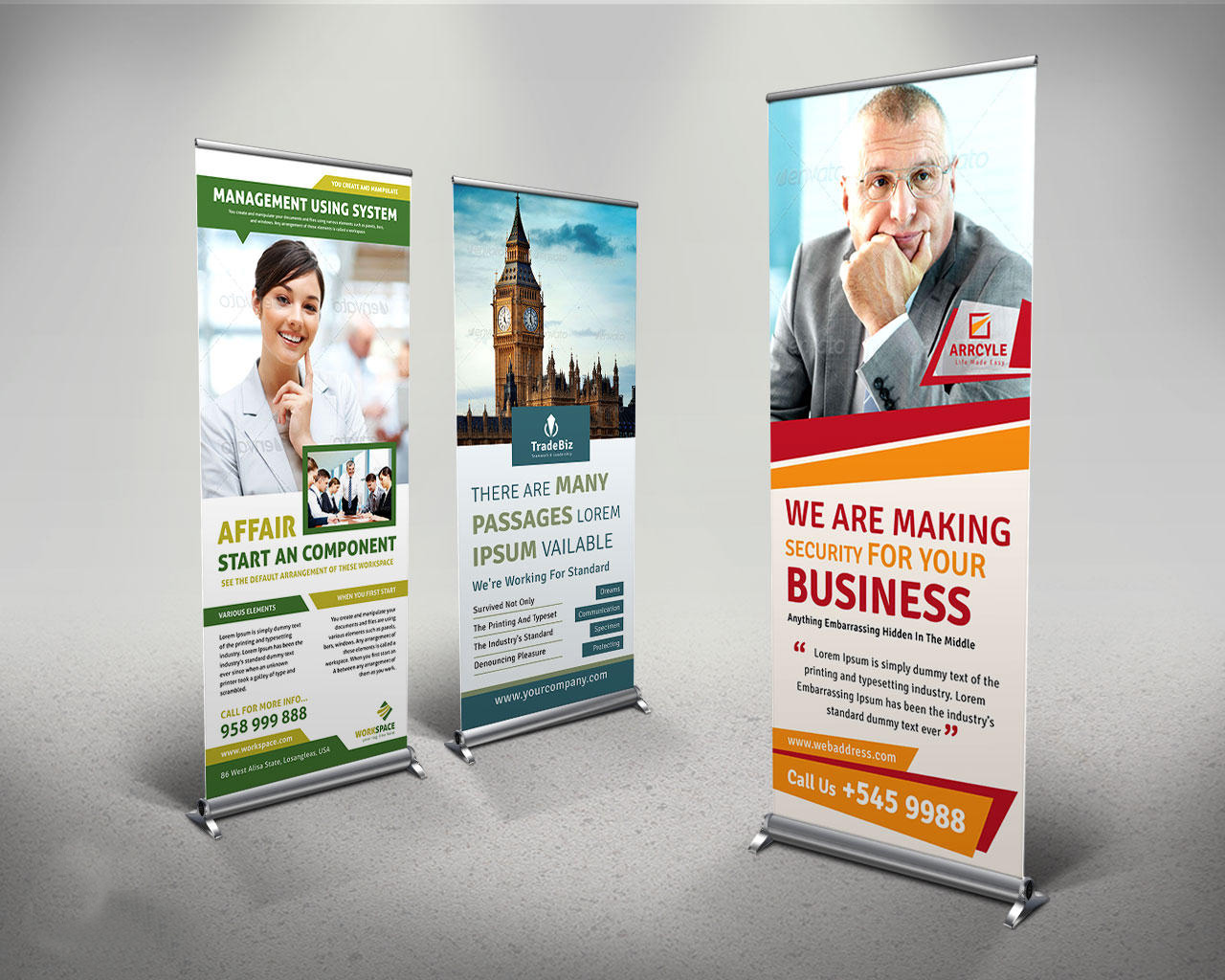The image portrays three floor-standing roll-up signs set against a clean, gray studio backdrop. These signs resemble the kind often seen at conferences or conventions.

On the far right, the first sign is vibrant in red and orange hues. It features a stern-looking Caucasian businessman with his hand on his chin. The text reads, "We are making security for your business," suggesting it promotes security services. At the very bottom, there is a contact number, 545-9988.

In the middle, the second sign prominently displays an image of Big Ben, the iconic London clock tower. The text on this blue-themed banner includes some placeholder text, reading, "There are many passages. Lorem Ipsum available. We’re working for standard." This appears to be a template design.

The sign on the left is green and yellow. It features a smiling woman, who seems to be wearing a lab coat, possibly indicating a medical profession. The text on this sign says, "Management Using System. A fair start component," along with a phone number, 958-999-888.

Overall, these signs appear to be sample advertisements showcasing different services and designs that a company might offer for various professional settings.